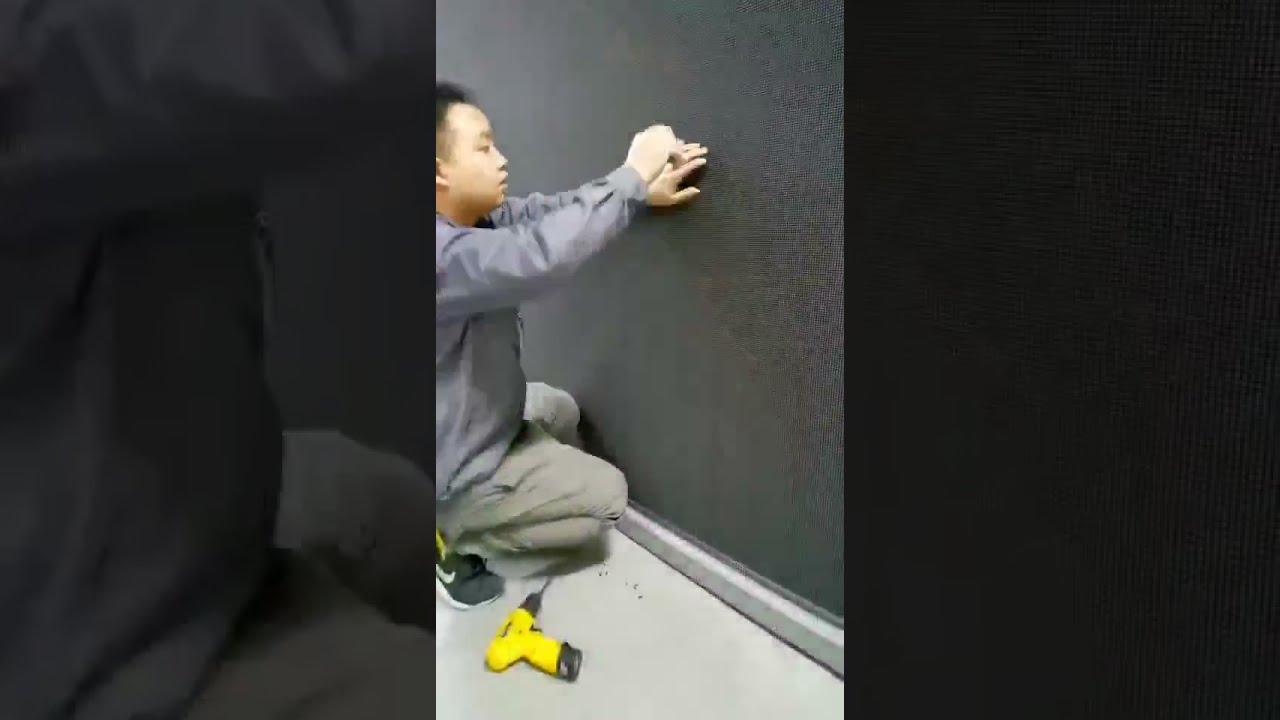The image is a horizontal rectangular photograph with grayed-out areas on either side framing a narrower rectangle in the middle. In the center, there is a man crouched down, working on a charcoal gray textured wall. He has both hands on the wall, with one hand over the other, as if trying to fasten or adjust something. A yellow power drill lies beside him on the light-colored floor. The man is dressed in khaki pants or possibly gray slacks, a blue or light-colored shirt, and black sneakers with a white Nike swoosh. He has short, dark hair and appears to be Asian. The grayed-out areas on the sides feature a blown-up, faded version of this image, with the left side showing a closer view of the man crouching and the right side being completely opaque. At the bottom of the wall, a baseboard is visible, adding a final touch to the indoor setting captured in this detailed photograph.